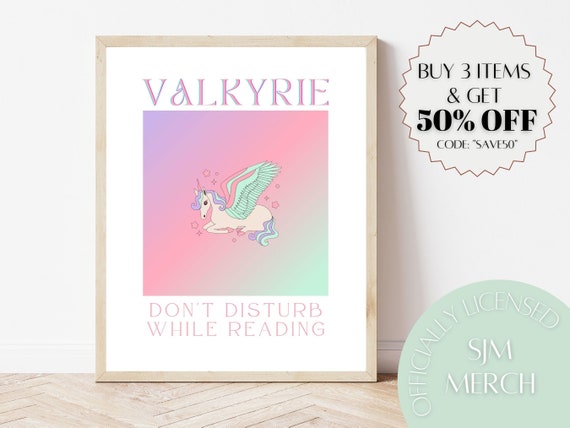The framed poster sits on a wooden floor, leaning against a white wall. Encased in a brown wooden frame, the poster features a white background with the word "Valkyrie" at the top in pink lettering. Beneath this, a square image showcases a Pegasus with turquoise wings, a blue-green mane, and a tail, lying down against a pastel backdrop of pink, light lavender, and green hues. Below the Pegasus, the text "Don't disturb while reading" is prominently displayed. In the upper-right corner, a circle with jagged edges states, "Buy three items and get 50% off. Code Save50." In the bottom-right corner, another green circle with white text reads, "Officially Licensed SJM Merchandise," indicating it is a product for sale. The overall composition conveys an advertisement for the item.